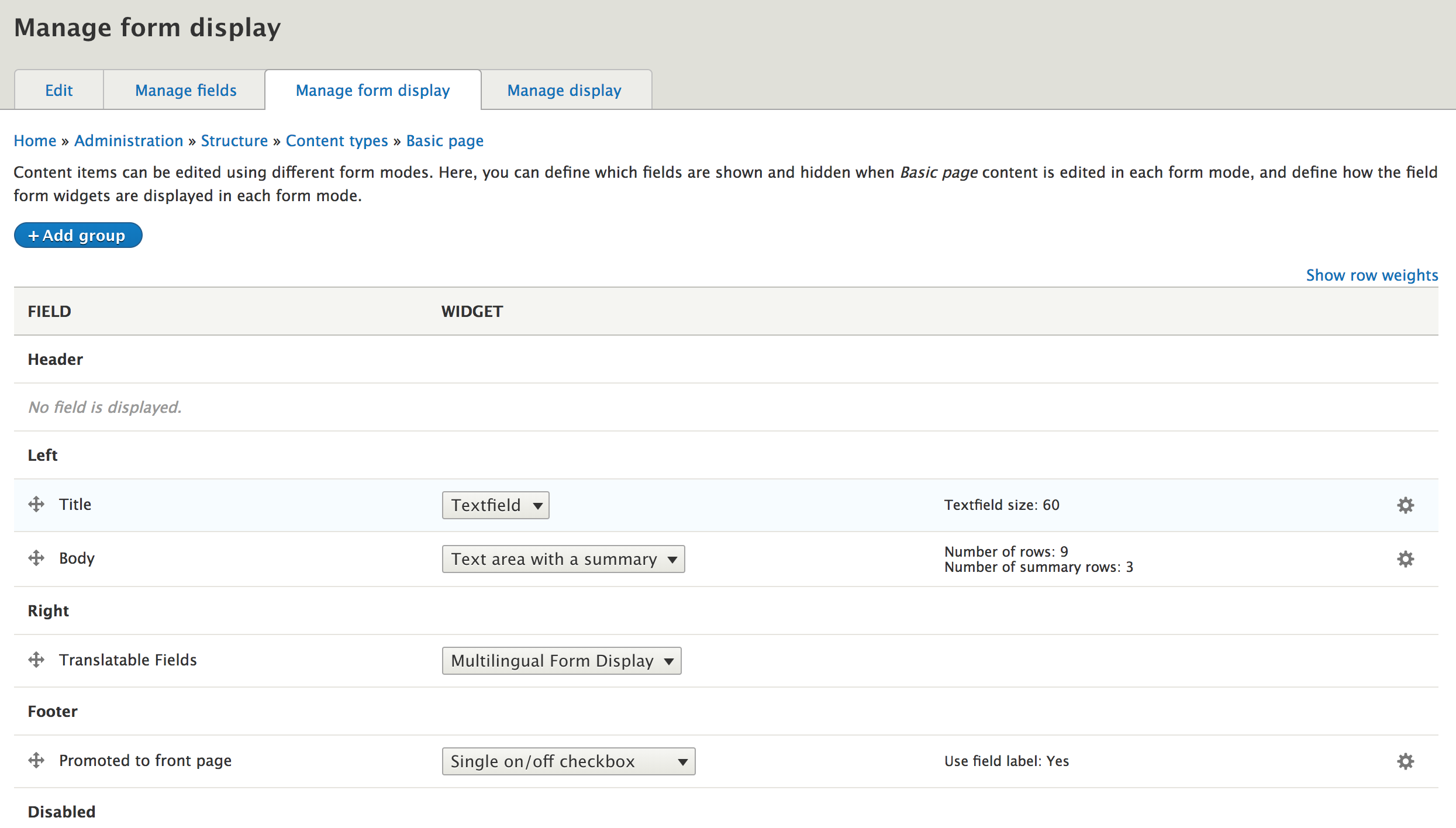The image is a screen capture showcasing a web interface for managing form displays. At the top of the image, a gray banner with black text reads "Manage Form Display." Below the banner, there are four rectangular boxes. Three of these boxes are gray with blue elements, while one is white with blue highlights. The first two gray boxes with blue text are labeled "Edit" and "Manage Fields." The third box, which is white with blue text, reads "Manage Form Display." The final gray box with blue text is labeled "Manage Display."

Moving down the image, there is a sequence of blue hyperlinked text that reads "Home," "Administration," "Structure," "Content Types," and "Basic Page." Further down, in black text, it states, "Content items can be edited using different form modes. Here you can define which fields are shown and hidden when basic page content is edited in each form mode and define how the field form widgets are displayed in each form mode."

A blue box follows, containing white text that says "Add Group," and includes a plus sign. Adjacent to it, in blue text, is "Show Row Weights." Below this, a gray box contains the headings "Field" and "Widget." Underneath the header "Field," it states, "No field is displayed," accompanied by a series of gray arrow icons.

The text continues with a list, starting with:
- "Left: Title, Text Field, Text Field Size 60, Cogwheel Setting."
- "Body: Text Area with a summary, Number of Rows 9, Number of Summary Rows 3, Cogwheel Setting."

Under the "Right" section it reads:
- "Translatable Fields, Multilingual Form Display."

In the "Footer" section, there are settings for:
- "Promoted to Front Page, Single Sign-On/Off Checkbox, Use Field Label Yes, Cogwheel Setting, Disabled."

Most of the above text and elements are displayed in various shades of gray, blending seamlessly into the interface design.